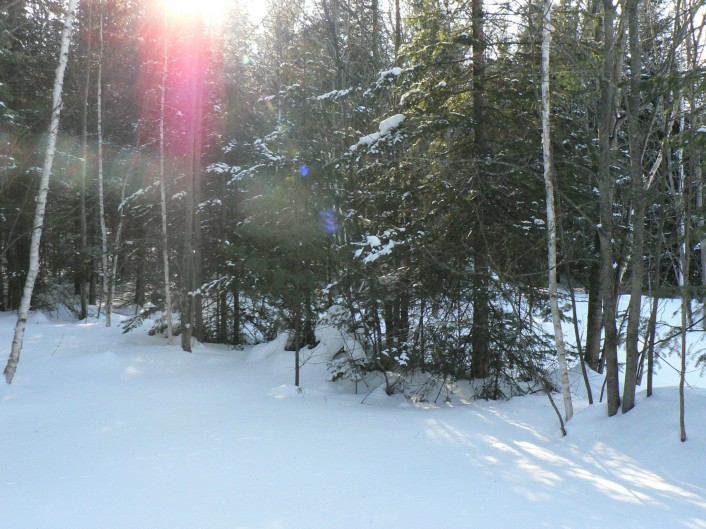The photograph captures a serene winter landscape within a forest, bathed in the soft glow of a late afternoon sun. The trees are predominantly barren, suggesting the cold grip of winter, with only the evergreen pines retaining small amounts of foliage. A thick layer of snow blankets the ground, approximately 6 to 7 inches deep, enveloping even some of the lower branches and trunks of the trees. The sunlight filters through the trees, creating a captivating interplay of pink and golden hues, especially prominent in the top left corner where the sun sits low in the sky. The sky, while mostly clear, has a muted, grayish tint. Among the trees, there are maples, oaks, and birches, identified by their distinctive bark and structure. The scene is tranquil, devoid of any animals or people, and appears untouched with a pristine, undisturbed layer of snow. This image, likely captured in a forest in North America or Europe, evokes the stillness and beauty of a winter day.